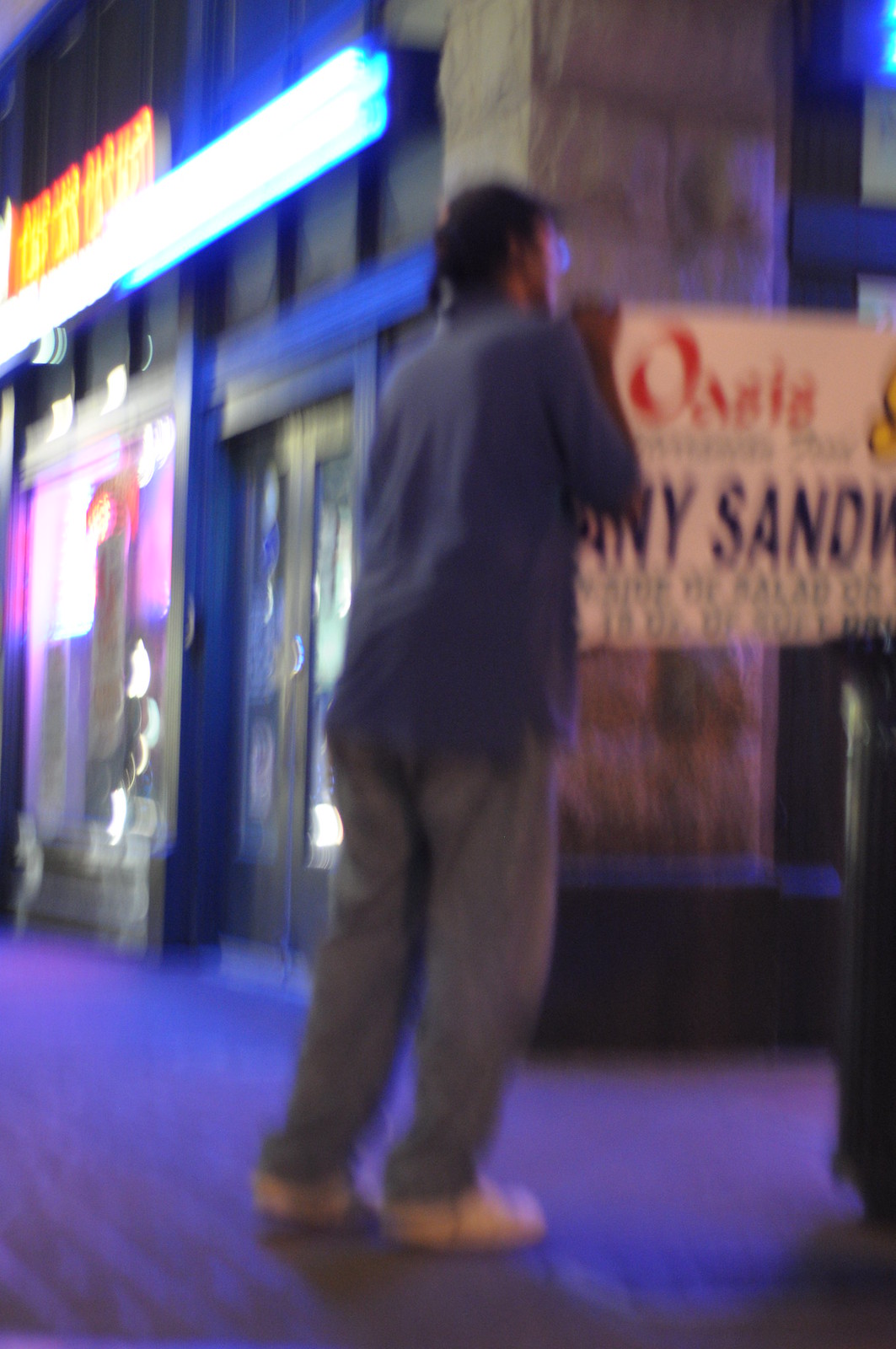In this blurry nighttime photograph, a man stands on the sidewalk outside an illuminated business establishment. The image, likely taken with a phone given its aspect ratio, centers on this man with his back to the camera, his figure dominating the frame. He has short black hair and appears to be Caucasian. He is dressed in a baggy, dark blue, long-sleeve button-up shirt that hangs loose over gray slacks or sweatpants, paired with white sneakers. 

The man’s stance is curious; he has his hands clasped and raised near his face, suggesting he might be wearing glasses, as evidenced by a faint blue reflection where his eyes would be. The background includes a glowing array of storefront windows and signs, casting a purplish hue onto the sidewalk. 

Notably, on the right side of the image and slightly above the man, there's a partially readable sign on a large concrete pillar that says, “Oasis” in red letters, hinting at the name of the establishment. Beneath it, fragments of words are visible, “Any” and “Sandwich,” suggesting the place might be a sandwich shop or restaurant. The street corner setting, with visible streetlights reflecting on the glass storefronts to the left, adds to the overall nocturnal ambiance of this scene.